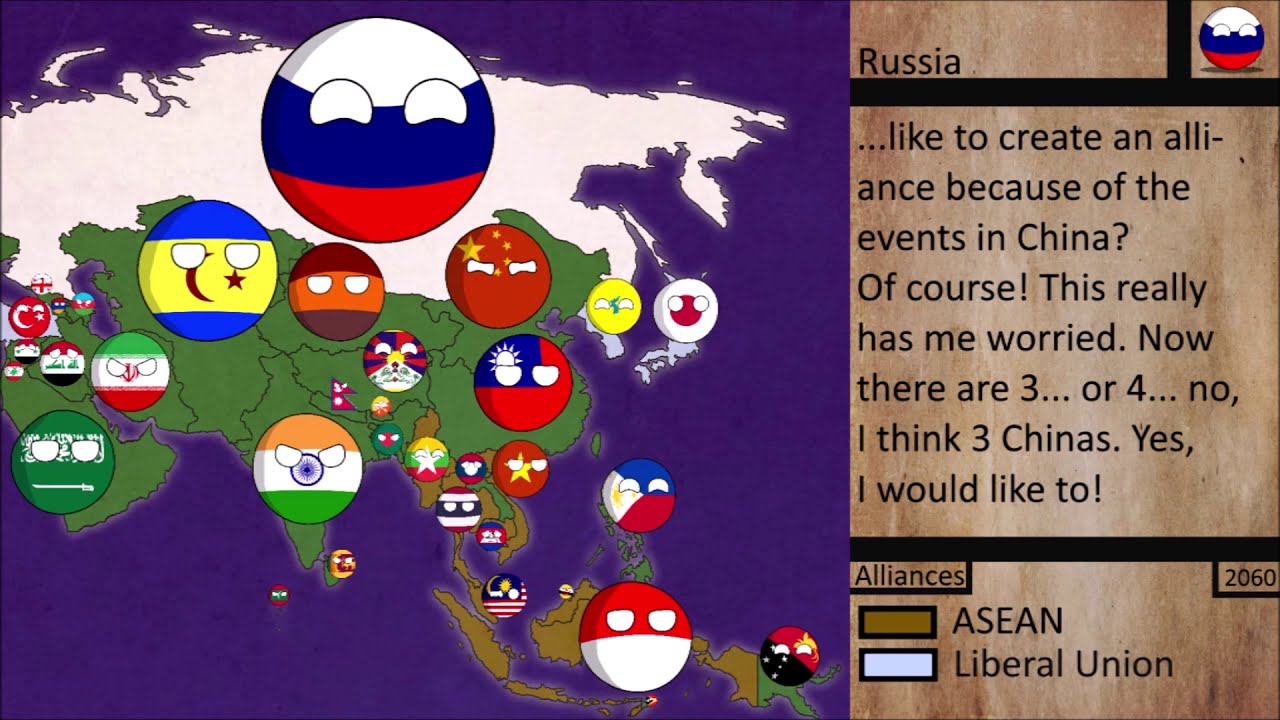The image depicts an interactive, cartoon-style learning game. It is split into two panels: the left panel covering about two-thirds of the image and the right panel taking up the remaining third. 

The left part of the image features a map with various regions outlined in different colors. The top part shows a white landmass likely representing Asia, while the bottom part depicts a green landmass, possibly Europe. Scattered across the map are numerous multicolored spherical avatars, each displaying the flag of a different nation, including China, Russia, Ireland, and Italy. These spheres are set against a dark purple background.

The right panel has a stone or kraft paper-like background sectioned off by bold black lines, resembling an Excel spreadsheet. At the top, it prominently displays the word "Russia." Below that, there's partially visible text that reads: "like to create an alliance because of the events in China?" This text is followed by a sequence of statements expressing concern about the situation in China and mentions of multiple "Chinas." Additional text at the bottom of this panel includes "alliances," "2060," "ASEAN," and "Liberal Union," with ASEAN in a brown box and Liberal Union in a white box.

Overall, the image combines both textual information and visual elements to represent geopolitical scenarios in an educational and engaging format.